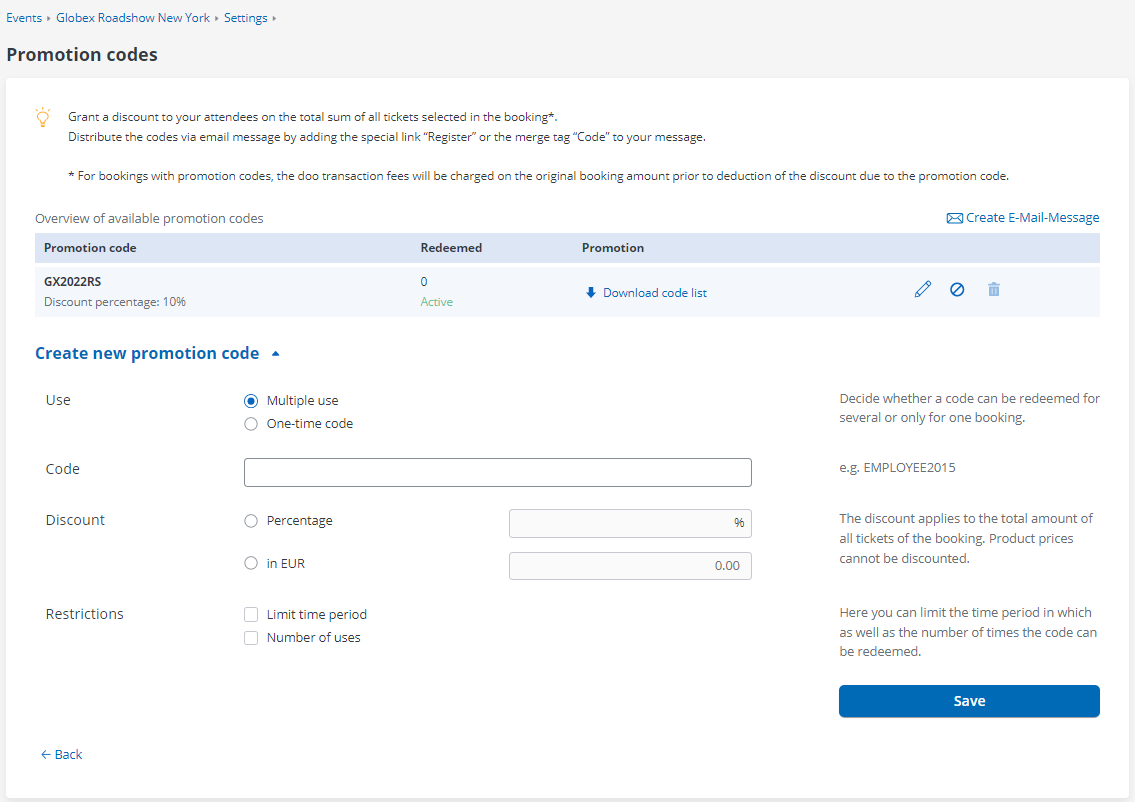**Caption:**

The image displays an interface for managing promotion codes. At the top of the screen, there are navigation tabs labeled "Events," "Globex Roadshow New York," and "Settings." Directly below this, the header reads "Promotion Codes," accompanied by an icon of a lightbulb emitting light, likely signifying an idea or important information. 

The main section provides detailed instructions on how to grant discounts to attendees based on the total amount of tickets selected during booking. It explains that the promotion codes should be distributed via email, using a special registration link integrated with the message through a merge tag code.

Further down, there is additional information about booking promotion codes and transaction fees. It states that transaction fees will be calculated based on the original booking amount before applying any discount from the promotion code.

There are also features allowing users to buy and send promotion codes or coupons. The transactions appear to be denominated in Euros. Users have the option to enter purchased codes into a designated field, and there's a downloadable code list available, suggesting that the cost of promotions might vary based on the downloaded content.

The background of the interface is white, with all text in black, ensuring clarity and readability. At the bottom, there's a prominent "Save" button for users to finalize their actions.